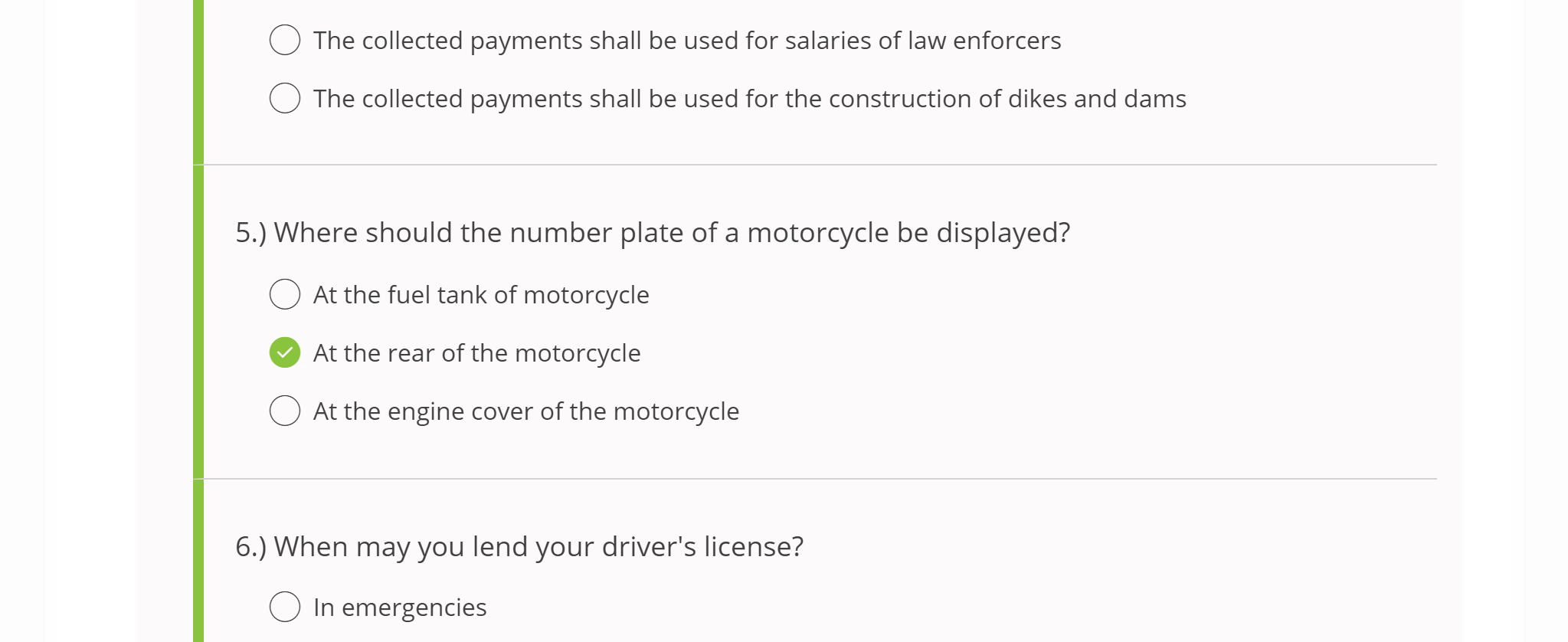This cropped screenshot depicts a segment of an online assessment, structured with questions vertically listed alongside corresponding answer options. Each question is distinctly numbered. Positioned centrally in the image is question number five, inquiring, "Where should the number plate of a motorcycle be displayed?" Three answer choices are provided, each accompanied by a selection bubble on the left: "at the fuel tank of a motorcycle," "at the rear of the motorcycle," and "at the engine cover of a motorcycle." The option "at the rear of the motorcycle" is selected. Furthermore, question number six is partially visible, asking, "When may you lend your driver's license?" with the sole visible answer option being "in emergencies," which remains unselected. The background of the interface is gray, adorned with a slim, green vertical line running along the left margin adjacent to the questions. Each question is demarcated by a delicate gray horizontal line. The upper portion of the screenshot reveals the bottom segments of the answer options for question four, though the actual question itself is obscured from view.